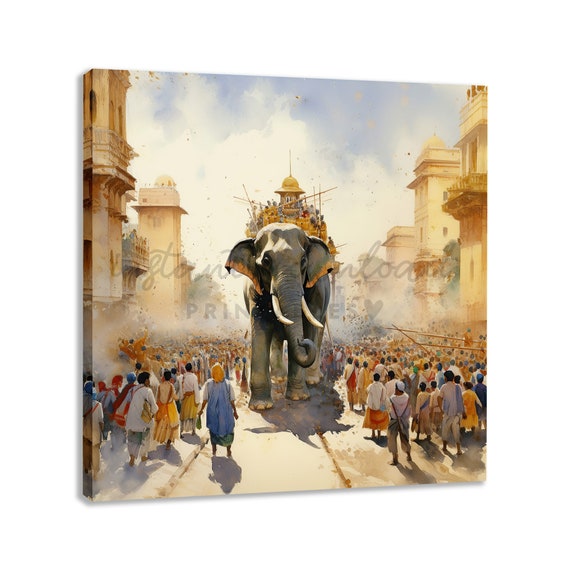In the heart of a bustling Middle Eastern or South Asian market street, a gargantuan elephant, estimated to be around 15 to 18 feet tall, strides majestically down a roadway tinged in yellow hues. The scene is a spectacle of culture and architecture, with towering, cream-colored buildings on either side of the street, their multi-story, rectangular forms made of sandstone-like material. Crowds of people, dressed in whites, blues, and yellows—many with robes and headdresses—throng the sides of the street, gazing up at the colossal creature.

The massive, gray elephant itself is adorned with an opulent structure atop its back, resembling a small, golden city or tower with a rounded dome, akin to a religious or cultural edifice; this intricate construction adds to the surreal and almost fantastical atmosphere of the scene. The elephant's long, pointed white tusks glint under the diffused light, which filters through a sky transitioning from brilliant blue to clouds and smoke.

A unique detail in the image is the indistinct watermark at the center, suggesting the image may be artistic or digitally created. The backdrop of light blue sky with clouds contrasts with the dense crowd and urban chaos below, while the elephant's imposing figure creates a swirling dust in its wake, adding to the dynamism of the street, alive with vibrant human activity and architectural grandeur.